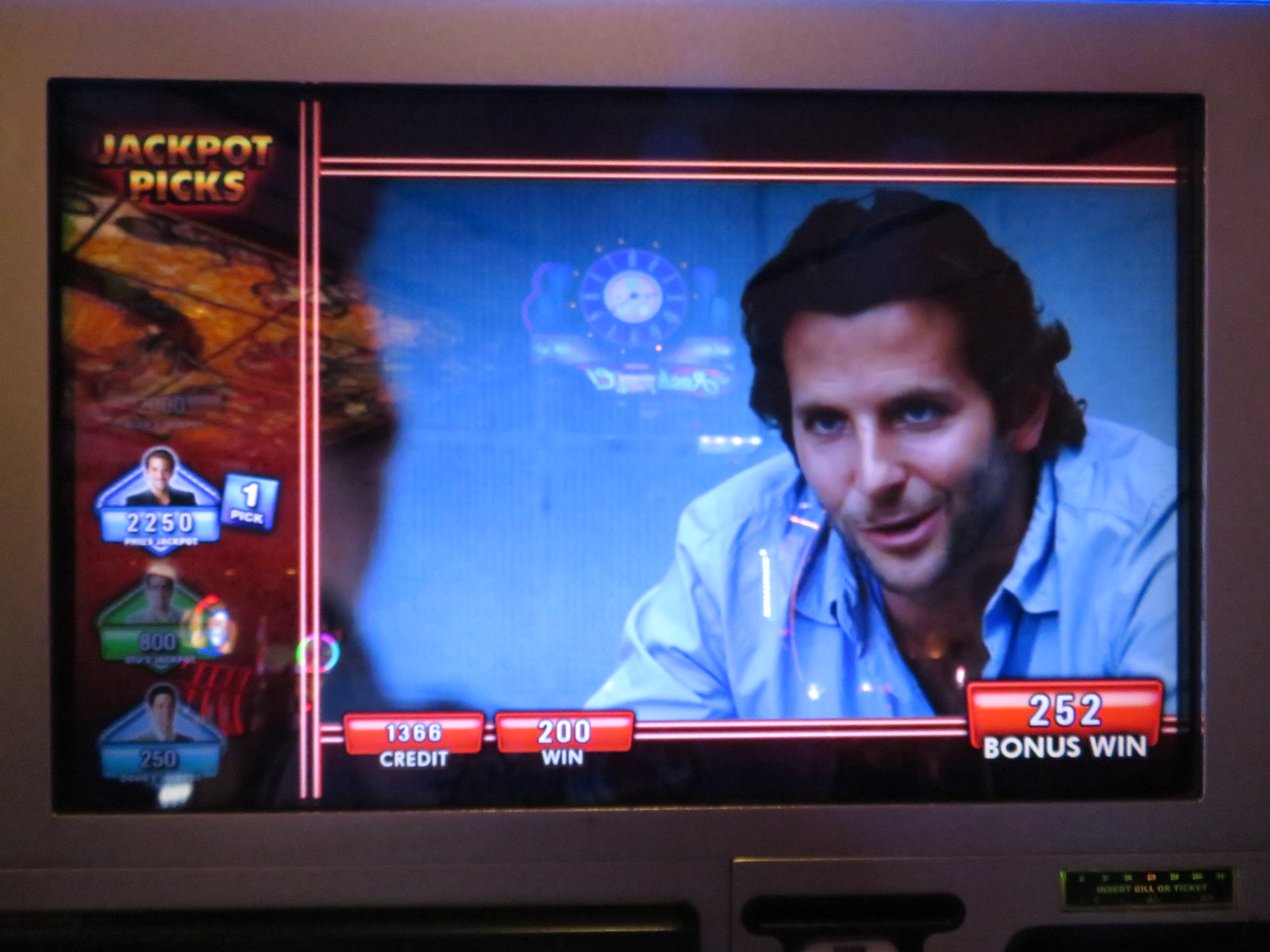The image is a detailed digital screenshot resembling a slot machine or gambling game, themed around the movie "The Hangover." Dominating the central part of the screen is a picture of Bradley Cooper's character from the movie, who is wearing a blue collared shirt. The background behind Cooper is also blue, while the overall background of the image is gray. To the left of Cooper's image, there is a section labeled "Jackpot Picks" in orange and yellow letters. Underneath this label, there are several smaller icons of different characters from the film, each with unique numbers beneath them, such as 2250.

At the bottom of the screen, there are statistics and buttons displayed in a red rectangular area: 1366 credits and 200 win, with a separate section to the lower right showing a bonus win of 252. This design suggests it might be a slot machine or gambling entertainment, possibly situated in a bar or a casino setting. The bottom edge of the image reveals black plastic inserts, indicating a slot or a place to insert a credit card, reinforcing the casino game atmosphere. Yellow and white text is used throughout the screen to highlight various pieces of information, creating a vivid and detailed visual connection to the gambling and entertainment theme of "The Hangover."